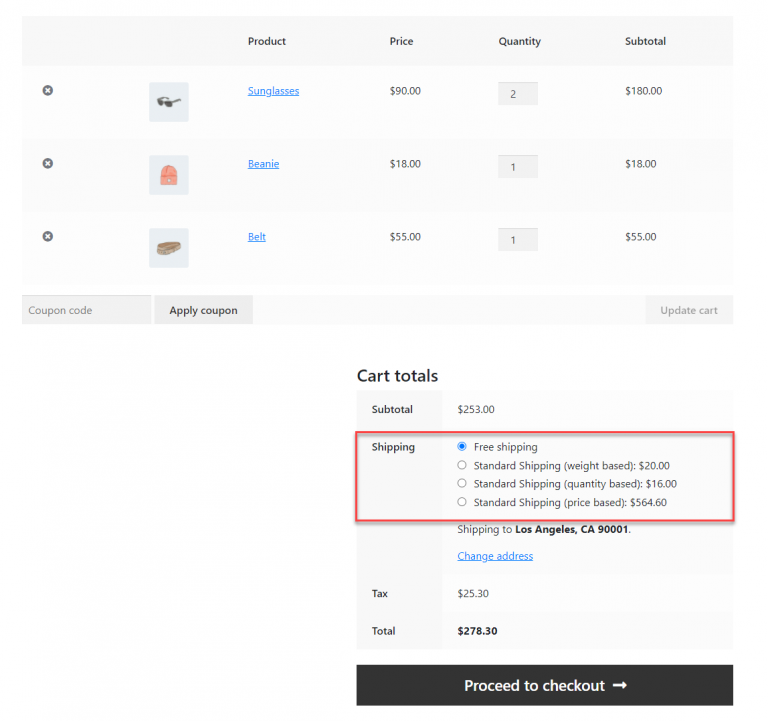This image depicts a cropped screenshot of a website's shopping cart interface with a grey background. At the top, a large grey banner spans the width of the screen, while a horizontal bar situated towards the right lists the headers "Categories," "Product," "Price," "Quantity," and "Subtotal" in bold black text.

Below this bar, three products are displayed, each accompanied by several details. To the left of each product entry is a grey circle containing an 'X,' which indicates an option to remove the item from the cart. Immediately to the right of this circle is a small square thumbnail image of the respective product. Aligned vertically under the "Product" header, the names of the products appear in a list. Corresponding prices are listed under the "Price" header, quantities under the "Quantity" header, and the subtotal for each item appears under the "Subtotal" header.

Beneath the list of items in the cart, the section "Cart Totals" is prominently displayed in large, bold black font. Within this section, a grey column on the left lists "Subtotal," "Shipping," "Tax," and "Total," each followed by the respective amounts on the right. The shipping options are highlighted with an edited red box, emphasizing that "Free Shipping" is selected. 

At the bottom right corner, a large black button labeled "Proceed to Checkout" invites the user to finalize their purchase.